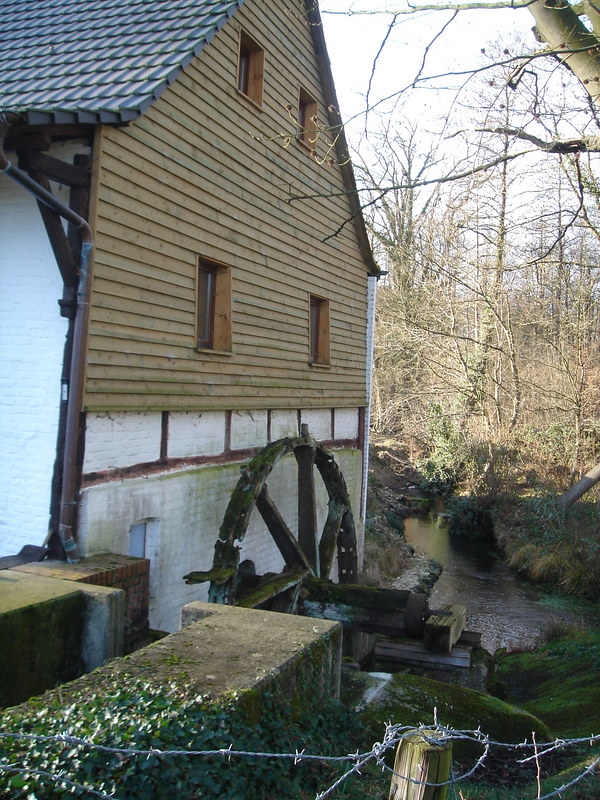The image depicts the side of an old mill, a three-story building with distinctive architectural details. The top half of the structure features wooden slats or shingle-like tiles, while the bottom half is constructed of white bricks, possibly stone. The roof is slate gray, adorned with small black squares. Prominently displayed on the lower side of the building is a large water wheel, positioned adjacent to a cement channel through which water flows. A slight waterfall can be observed, enhancing the rustic and historic charm of the mill. The foreground includes a fence post with barbed wire, suggesting restricted access to certain areas. Moss-covered stone walls are visible at the bottom right of the house, in the lower left corner of the image's perspective. In the background, a dense wooded area lines the riverbank, contributing to the serene outdoor setting, which appears to be bathed in daylight. The scene features a palette of tan, brown, green, white, and slate gray tones, evoking a tranquil yet industrious atmosphere.